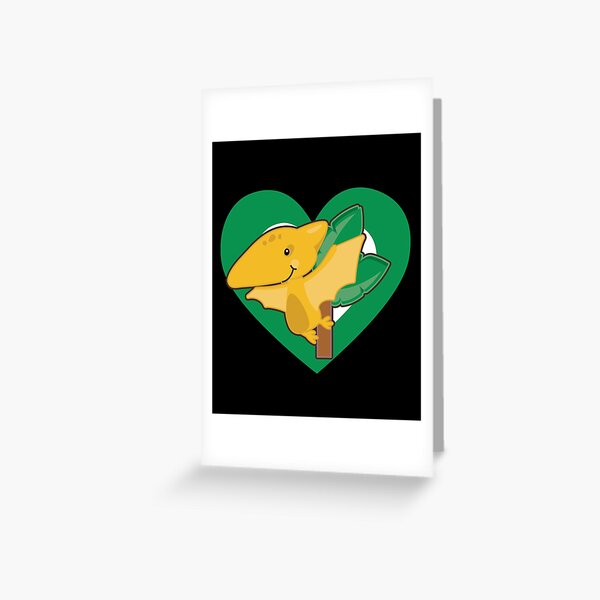This image features a prominently centered, Polaroid-style photo set against a stark white canvas wall. The main focus, housed within a rectangular white background, is a black square. Inside this black square lies a green heart with a slight white gradient in the center. The heart frames a whimsical, cartoonish scene. Dominating the scene is a gold-headed, yellow pterodactyl with a cheerful expression, marked by black eyes and a black outline. Its lighter yellow wings are spread wide, and it boasts a brownish mustard belly. This enchanting creature appears to have spots of the same darker hue around its face. Behind the pterodactyl stands a stylized palm tree, characterized by a slender brown trunk and green leaves, both of which continue the fantasy cartoon theme. This entire setup gives the impression of a playful, child-like drawing with no additional colors apart from variants of white, black, green, yellow, and brown, and without any accompanying text. The overall impression evokes a sense of innocence and imagination.